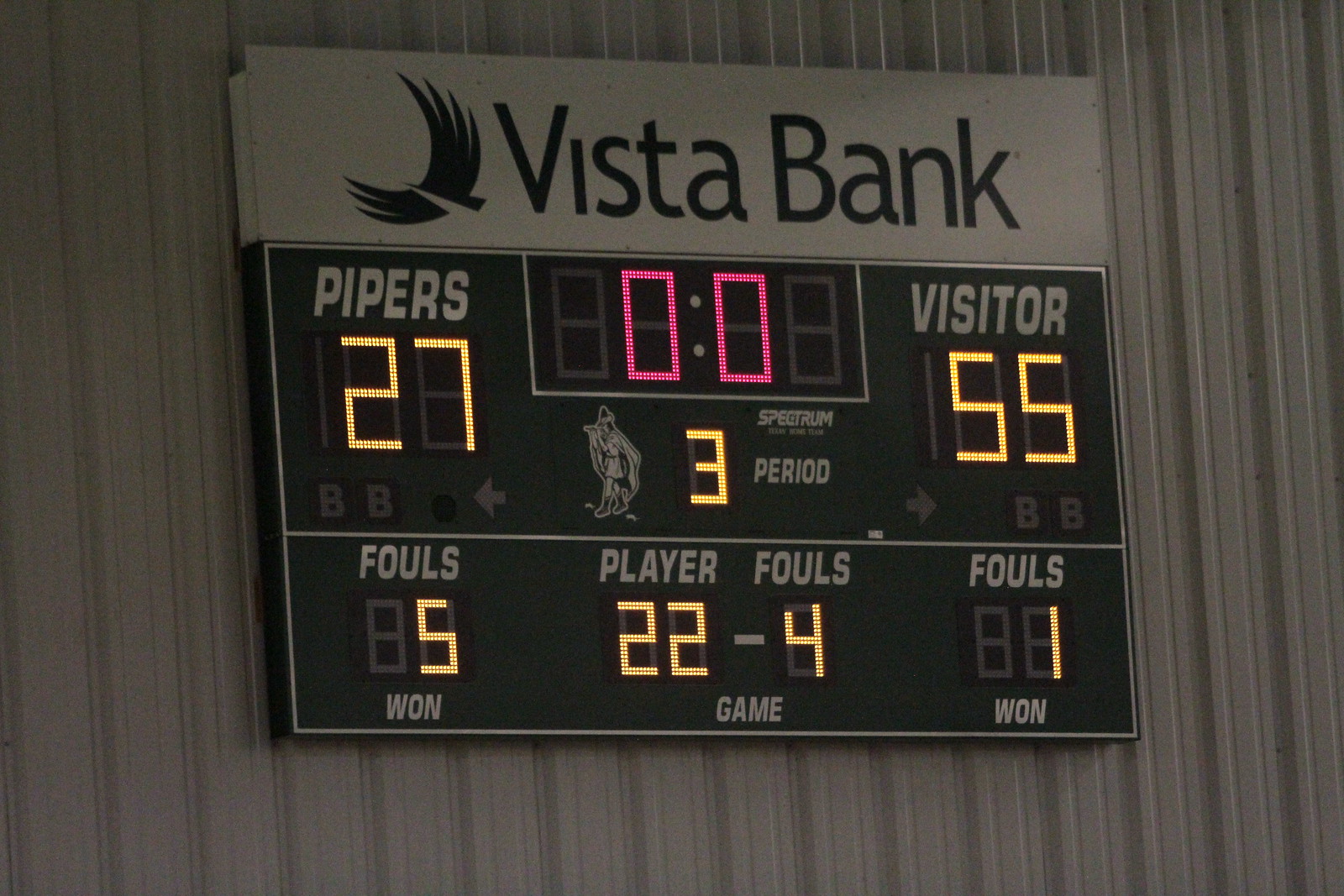This detailed photograph captures a dark green rectangular scoreboard mounted on a white, sheet-metal wall with vertical lines. At the top, the board features the name "Vista Bank." Below that, centrally located, a digital LED display shows the timer reading "00" in pink. Beneath this timer, another LED display indicates that it is the 3rd period. The scoreboard is divided into sections to display various game statistics.

On the left side, under the label "Pipers," an LED screen displays the score "27." To the right, under the label "Visitor," another LED screen shows the score "55," making the score 27 to 55 in favor of the visitors.

A white horizontal line separates the upper and lower sections of the board. Below this line, on the left side, there is an LED display showing "5" for "Fouls" with a small "1" beneath it. In the middle section, under "Player Fouls," another LED screen reads "22-4" for player statistics, with the word "Game" directly below. On the right side, under another "Fouls" label, an LED display shows "1," with another "1" directly beneath it, correlating with the previous foul count.

The combined LED displays use yellow and red colors to convey their numbers and information, ensuring clear visibility of all game statistics.